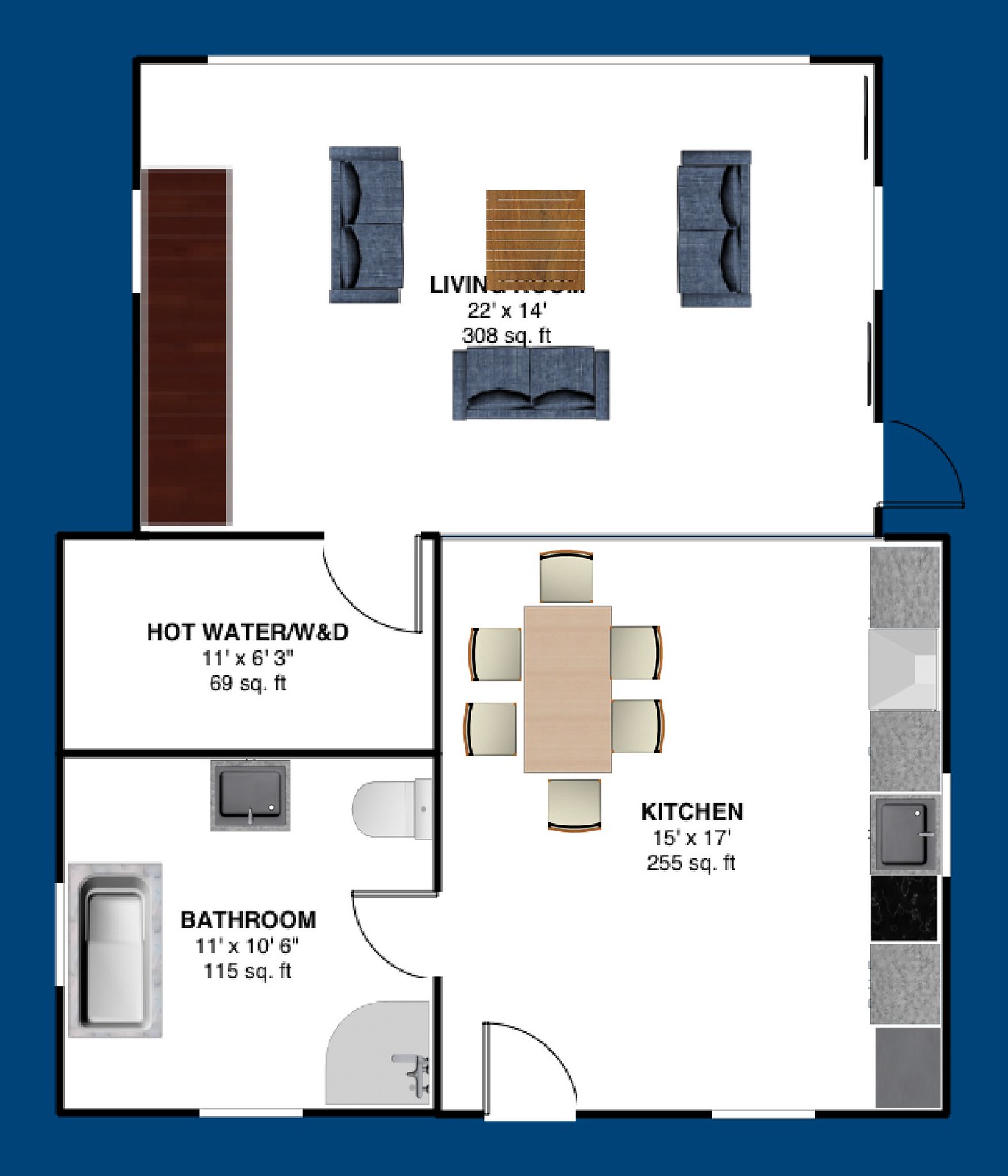Blueprint for a Home's First Floor

A detailed floor plan for a home is depicted on a dark navy blue background. The layout meticulously outlines each room with measurements. 

- **Living Room:** Located at the top of the blueprint, this room is labeled “Living” (partially covered) and measures 22 by 14 feet, amounting to 308 square feet. It is furnished with three loveseats or two-seated couches arranged around a central coffee table.
  
- **Hot Water Closet:** Adjacent to the living room, this utility space is labeled “Hot Water WND” and measures 11 by 6.3 feet, totaling 69 square feet. 

- **Bathroom:** Next to the hot water closet, the bathroom measures 11 by 10.6 feet or 115 square feet. The layout includes a bathtub, sink, toilet, and possibly a shower stall. 

- **Dining Room:** Measuring 15 by 17 feet and totaling 255 square feet, the dining room features a long table with seating arranged as follows: two chairs on the longer side and one chair at each head of the table. 

This thorough and carefully structured floor plan offers a glimpse into the functional and spacious design of the home's first floor.